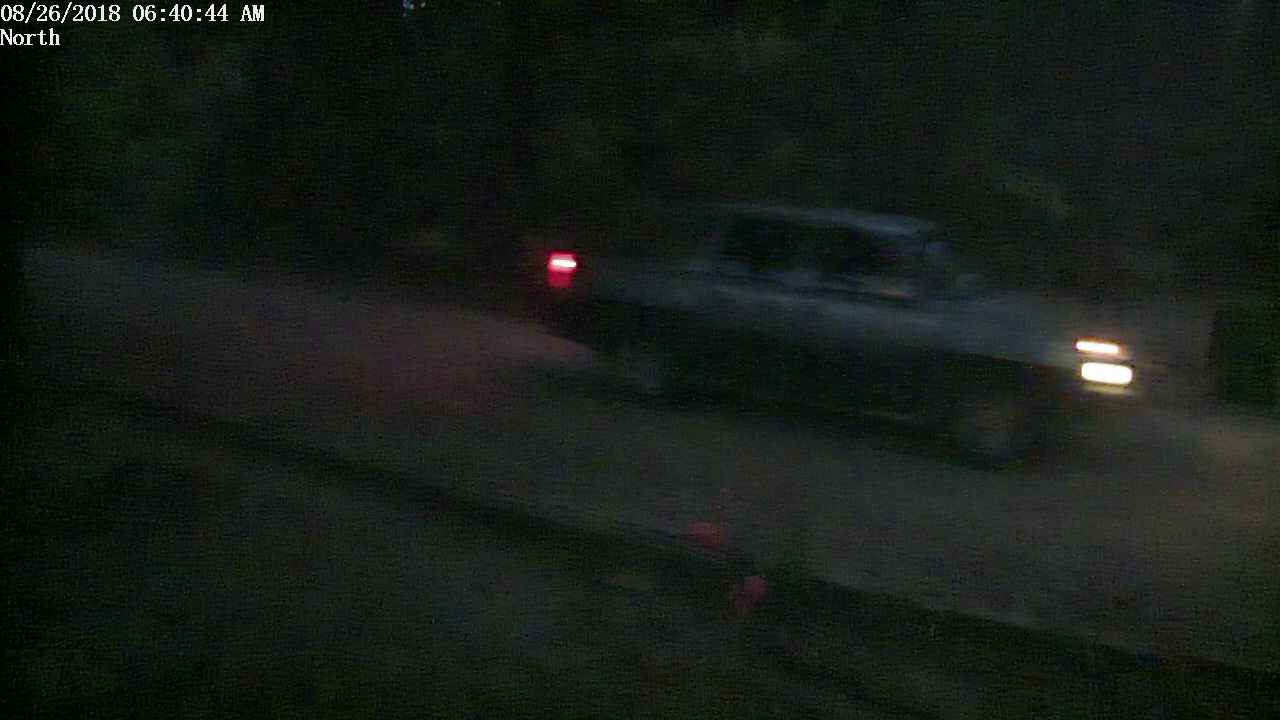In this nighttime photograph, captured by a low-quality security camera, a grayish, squarish SUV is seen driving on a slightly tilted, possibly raised, gray road that resembles a sidewalk. The road runs from the top left to the bottom right of the image. The SUV, with its headlights and brake lights illuminated, appears to be heading to the right. The vehicle's right side, which includes larger rear passenger windows, is more visible, suggesting it might be a four-door model. The background hints at a forest-like area, with indistinct trees creating a dark, blurred backdrop. Overlaid in white, computer-generated text at the top left corner reads "08/26/2018," "06:40:44 a.m.," and "North," marking the date, time, and direction of the scene.